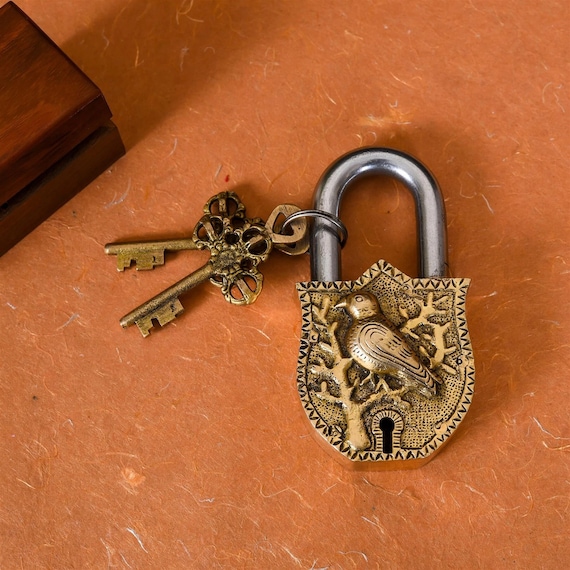This detailed close-up photograph showcases a staged scene of a decorative, antique-like brass lock and intricate keys, situated on an orange background. The padlock, predominantly gold with a silver top, features an ornate design with a large bird etched onto a tree. The bird and tree design envelops the keyhole, which has a dark, decorative pattern surrounding it. The keys, designed to mirror an old-fashioned aesthetic, are attached to the lock by a small loop, enhancing their antique appearance. In the upper left-hand corner, a small brown wooden box is partially visible, adding to the vintage feel of the composition. Despite its convincing antiquated design, the setup appears too deliberate, suggesting that both the lock and keys are modern creations made to look antique.